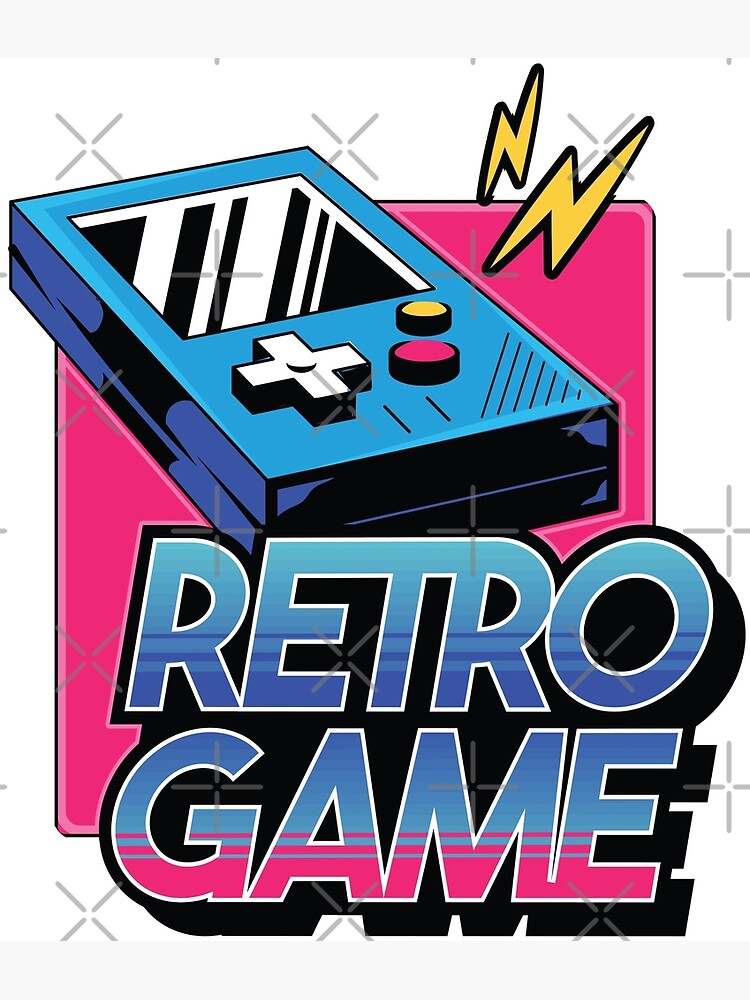This illustration depicts a retro-style handheld gaming device reminiscent of a Game Boy, rendered in cartoon format. The device is blue, rectangular in shape, with a white directional pad on the left and two circular buttons—one pink and one yellow—on the right. Above the buttons is a small screen that occupies nearly half of the device's front. Surrounding the gaming device is a vivid pink square background. Below it, the text "Retro Game" is prominently displayed in blue and pink with horizontal striping. Accentuating the dynamic feel of the image, two yellow lightning bolts emerge from the top of the device. The image also features a pattern of translucent gray crosses and pluses scattered throughout the white background, reminiscent of a watermark.